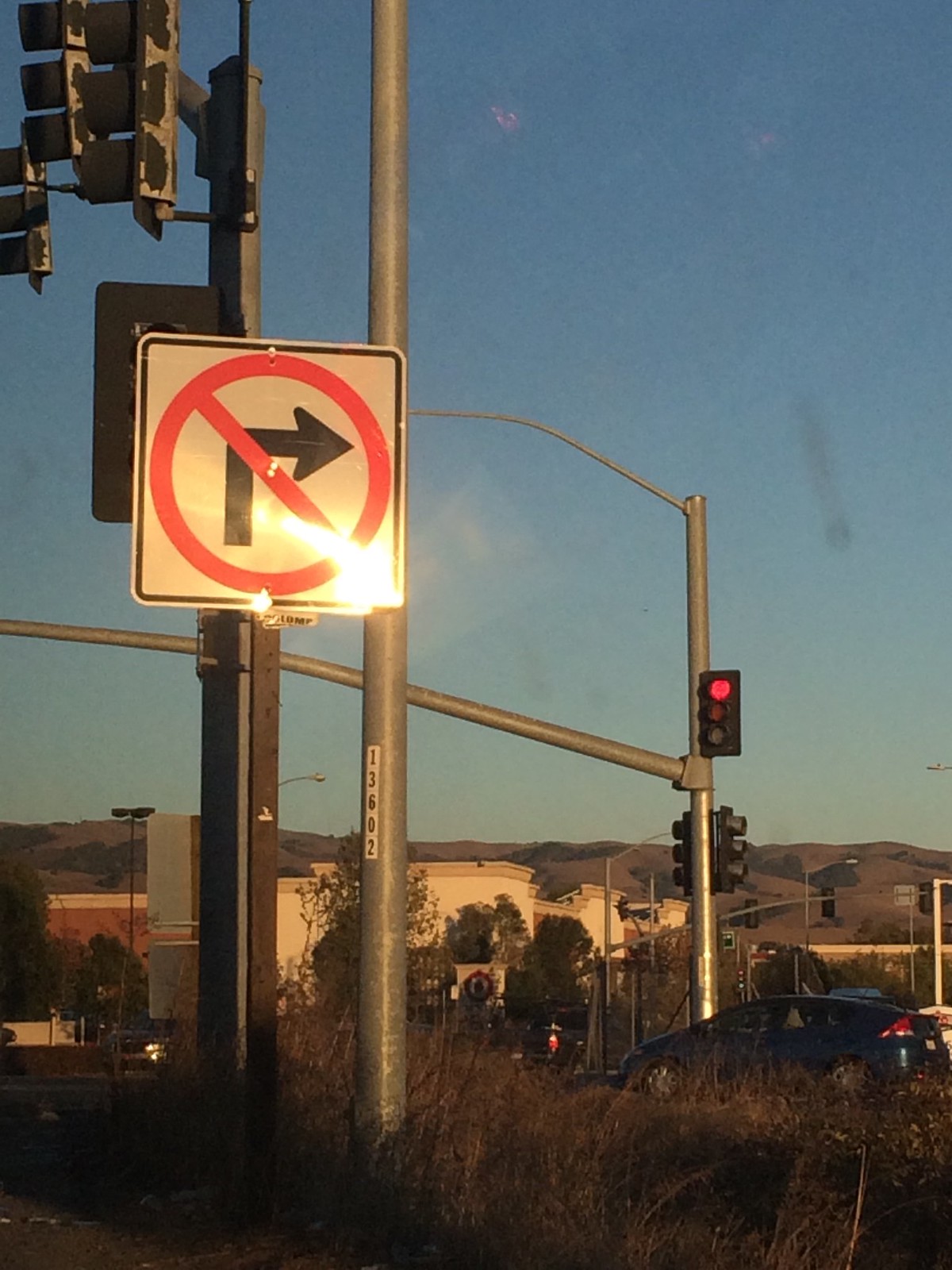The photograph is a rectangular image with longer sides on the left and right, capturing a clear, light blue sky with no clouds, tinted in an orangish-yellow hue that suggests the sun is setting. In the foreground, tall, brown grass grows at the very bottom, partially obscuring a large metal pole with the number 13602 on it. Next to this pole stands a square-shaped pole with a street sign, predominantly featuring a white background with a black border. This sign displays a right-pointing arrow with a red circle and diagonal line, indicating no right turn. The pole is round and supports the traffic sign, while additional traffic lights are positioned above the scene, one of which faces the camera with a red light. 

In the background, a clear sky stretches out, revealing the ridges of a mountain range and a collection of buildings that appear to be part of a shopping center complex. A blue car, likely a commuter vehicle, and a black car can be seen on the street below the signage. Sunlight reflects off nearby metal signs, reinforcing the impression of dusk.